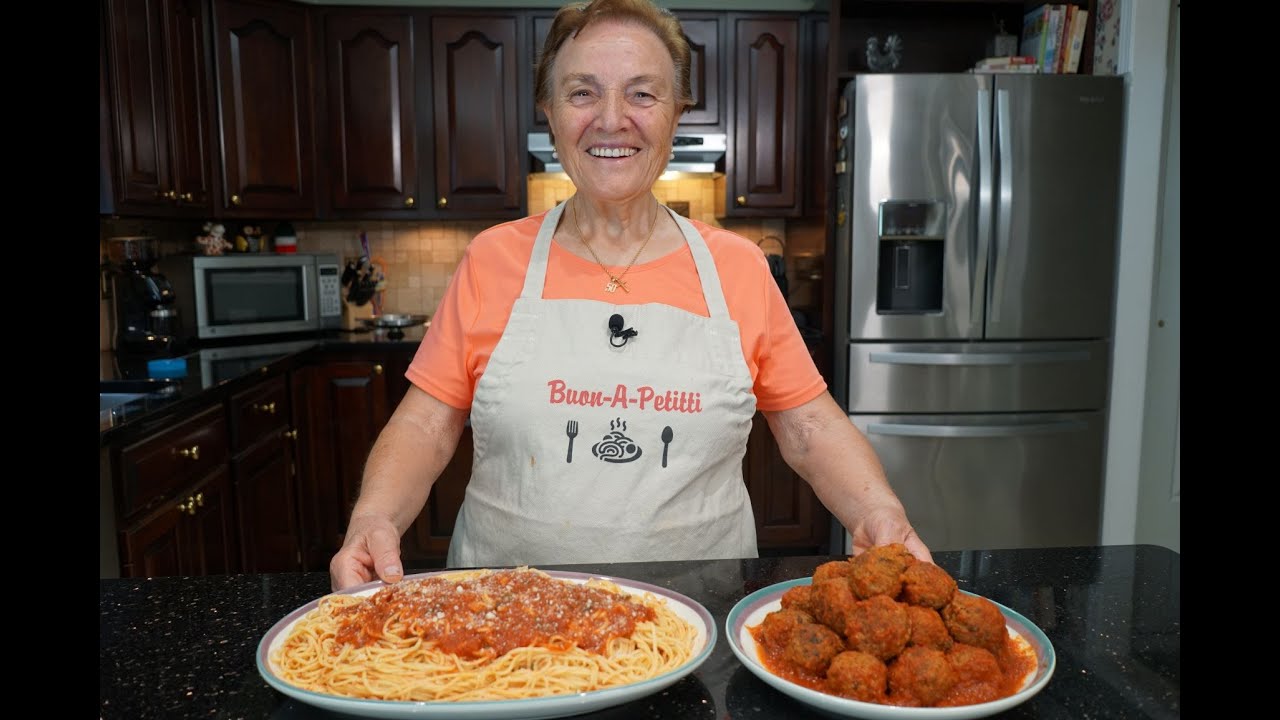In this photorealistic image, an older Caucasian woman with brown hair tied back is standing behind a black granite countertop in a kitchen. She is smiling warmly at the camera, wearing an orange t-shirt and a white apron that says "Buon Appetito" in red writing, adorned with a cartoon rendition of a fork, knife, and a plate of pasta and meatballs beneath it in black. A gold necklace and a clipped-on microphone suggest she might be recording a cooking show.

On the countertop in front of her rest two plates. The one on the left is a large, oval-shaped white plate with a blue rim, laden with a generous heap of golden spaghetti topped with rich tomato sauce and a sprinkle of white parmesan cheese. The plate on the right, circular and matching in design, showcases a pyramid-like stack of meatballs smothered in red sauce. She holds each plate with one hand.

The kitchen in the background features dark brown, possibly cherry wood cabinets, both upper and lower, with black countertops and a brownstone backsplash. A silver microwave sits in the corner on the left side, while a stainless steel refrigerator is visible on the right. The overall composition is wide, filling the frame horizontally to reveal the immaculate and warmly lit kitchen setting.